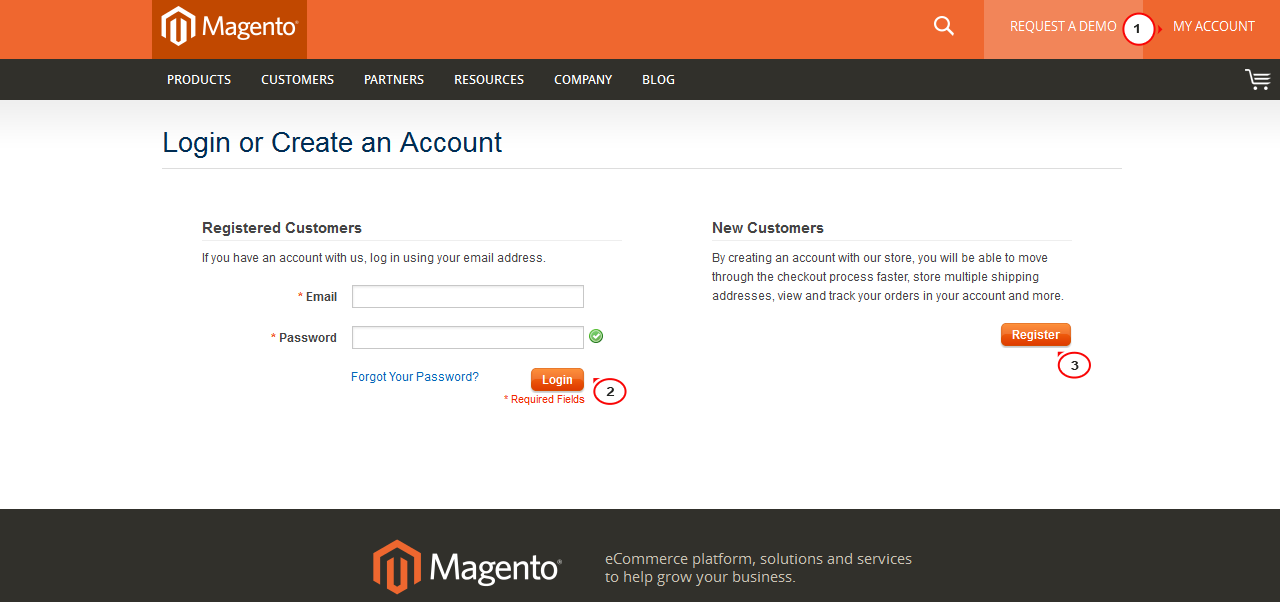This screenshot captures the login page of the Magento website. At the top, there's an orange header featuring the Magento logo on the left. On the right side of this orange header, you'll find a search icon, a button to request a demo, and options to access 'My Account', highlighted by a red circle with the number '1'.

Below this orange section is a black navigation bar with clickable options, including Products, Customers, Partners, Resources, Company, and Blog. 

Directly beneath this black bar is a white background section divided into two main areas. On the left, under 'Registered Customers', the page prompts users to log in with their email and password. It includes input fields labeled 'email' and 'password', a 'Forgot Your Password' link, and a 'Log In' button. The 'Log In' button is marked with a red circle containing the number '2'. 

To the right, in the 'New Customers' section, the website highlights the benefits of creating an account, such as faster checkout, storing multiple shipping addresses, and tracking orders. A 'Register' button is accessible here, also marked by a red circle with the number '3'.

Finally, at the bottom of the page, there's another black section reiterating the Magento brand and its tagline: "e-commerce platform solutions and services to help you grow your business."